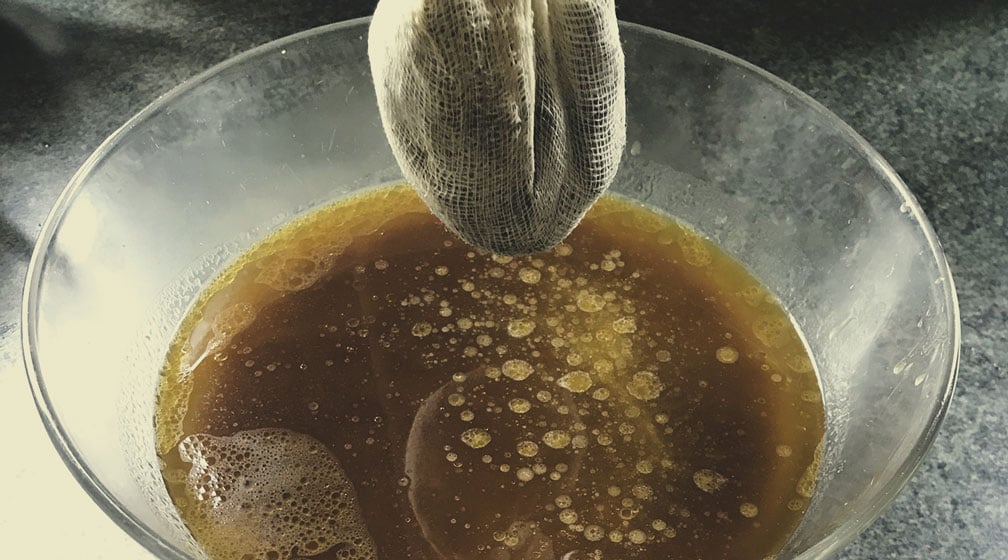The image showcases a clear, wide glass bowl filled with a brownish liquid that exhibits a greasy, oily appearance with lighter brown spots, golden bubbles, and some white foam floating on the surface. The bowl is resting on a gray, granite-like countertop. Above the bowl is a white mesh or cheesecloth bag filled with an unidentified black substance, appearing as if being dipped into the liquid to infuse or flavor it. The liquid could potentially be tea or a type of broth, given the presence of the dipping bag and the described appearance of both the liquid and the cloth. The scene has a slightly foggy ambiance around the bowl, emphasizing the details within the bowl and the infusion process taking place.